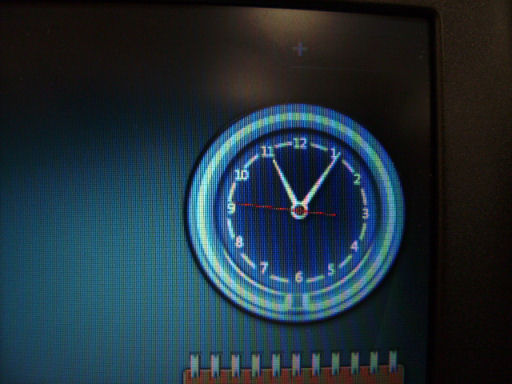The image showcases the right side of a computer monitor or television screen, displaying a computer-generated or animated clock. The clock face is blue, featuring white hour and minute hands, and a distinct red seconds hand. Below the clock, there is a digital spiral graphic. Another spiral, reminiscent of a metal coil from an orange notebook, is visible at the top of the screen, with the orange color distinctly seen through the coil. The digital nature of the image introduces red and blue lines across the screen, likely due to the capture method. In the background, to the right of the monitor, a black wall can be observed.